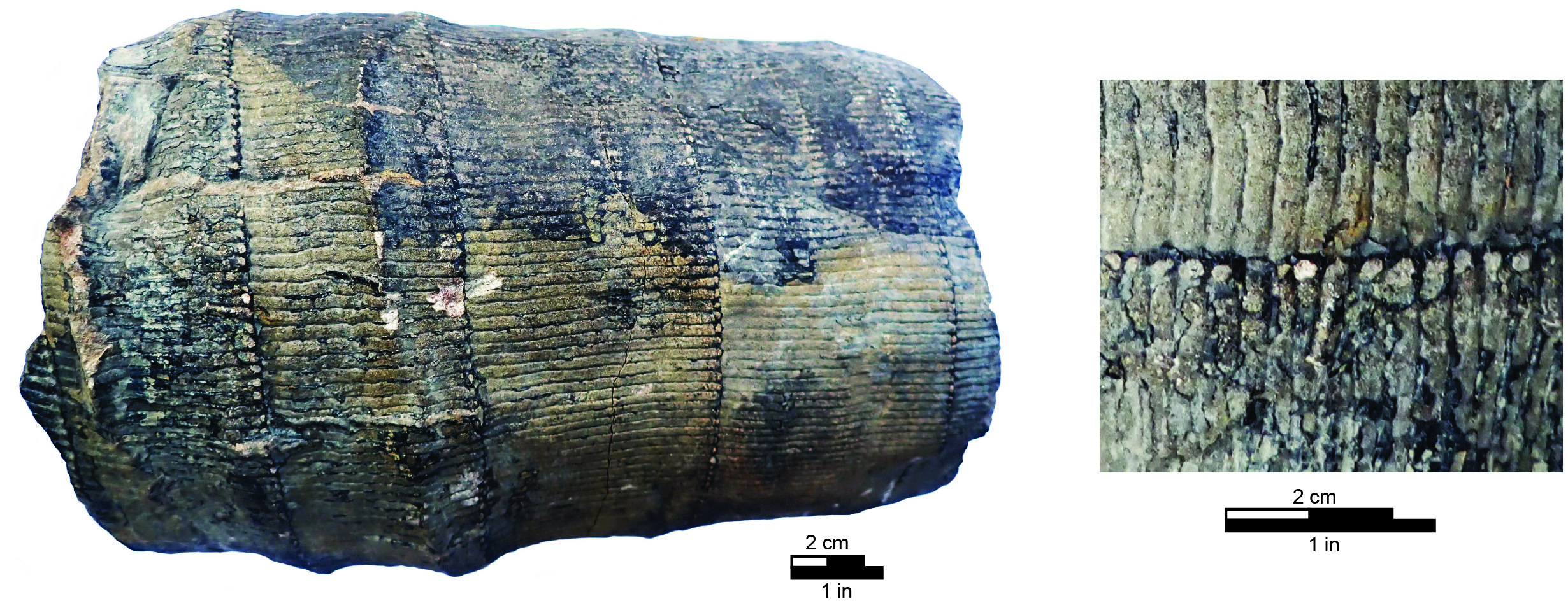The image features a large, cylindrical fossil on the left, likely a calamite, characterized by its potato-like round shape and ragged, rocky surface. The fossil displays a distinctive texture with horizontal, rectangular scales and striations running between the scales. Its coloration transitions from a tan or golden-yellow at the lower half to a dark gray with light gray splotches at the top. Below this fossil, there is a scale indicator that represents measurements in both inches and centimeters, suggesting an approximate size of around 12 inches in circumference.

To the right, an inset photo provides a close-up view of the fossil's scales, accentuating the rough and rocky texture. This inset photo also features a scale with measurements in centimeters and inches. Both images are set against a white background, allowing the intricate details and varying shades of browns, tans, blacks, and hints of blue to stand out prominently.